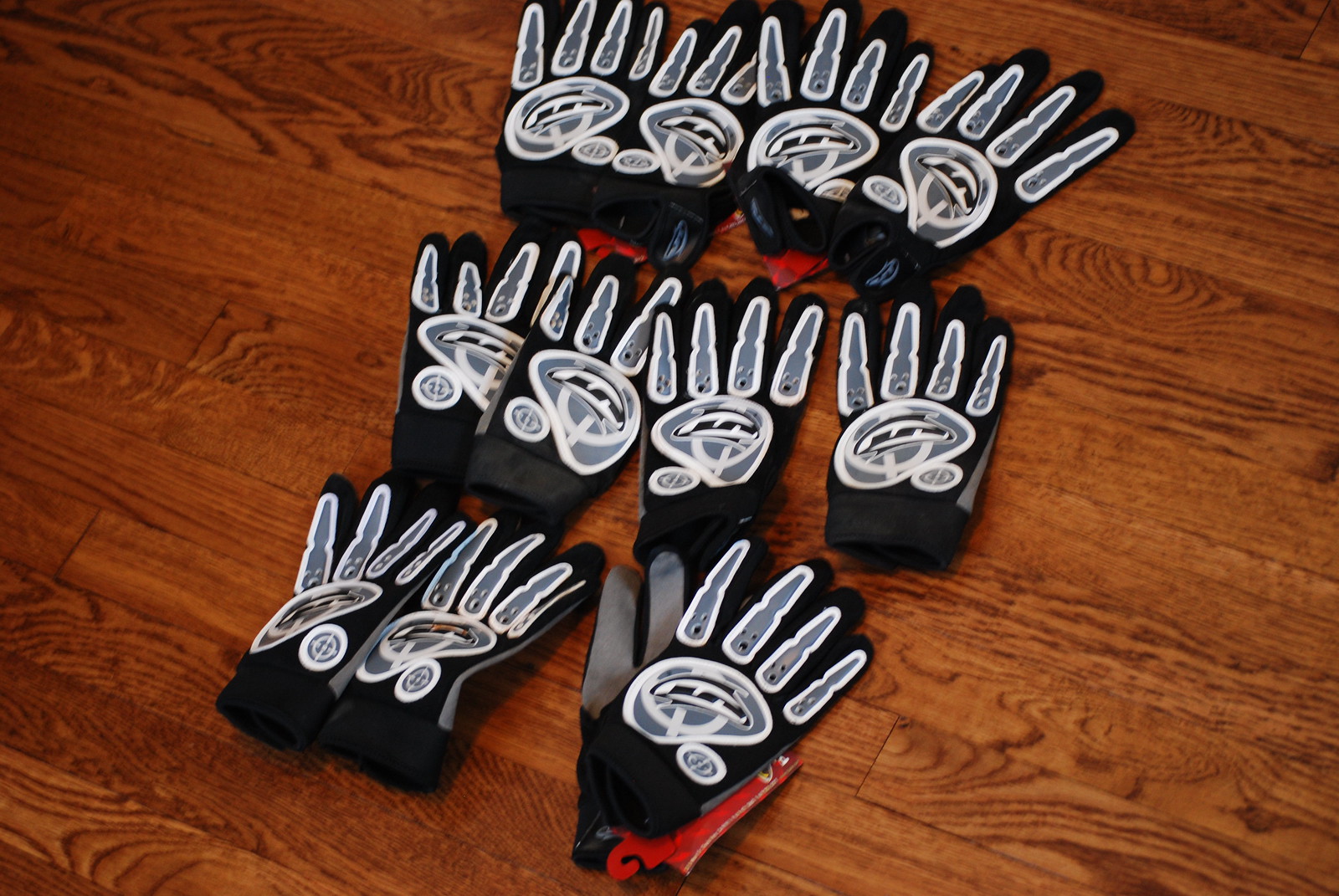This horizontal rectangular photograph features six pairs of black gloves meticulously placed on a brown wooden surface with visible knots. The gloves are arranged in three rows, with two pairs in each row, slightly offset diagonally from the top right to the bottom left. The pairs on the top row and middle row show the back of the gloves, while in the bottom row, one pair has gloves positioned with one facing up and the other showing the palm side.

These gloves are distinguished by skeletal designs on the fingers—gray on the inside with white outlines—reminiscent of bones. Each glove prominently displays a round, dual-logo near the wrist; the main logo is centered with a smaller one at its bottom right. One glove in the bottom row features a visible red clip, indicating it's probably part of a retail display, possibly attached to a hidden price tag. 

The wooden surface, evident from the medium stain and plank size, likely suggests it's a brown table or floor. The detailed arrangement and distinct skeleton motif on the gloves make this image visually striking and methodically detailed.